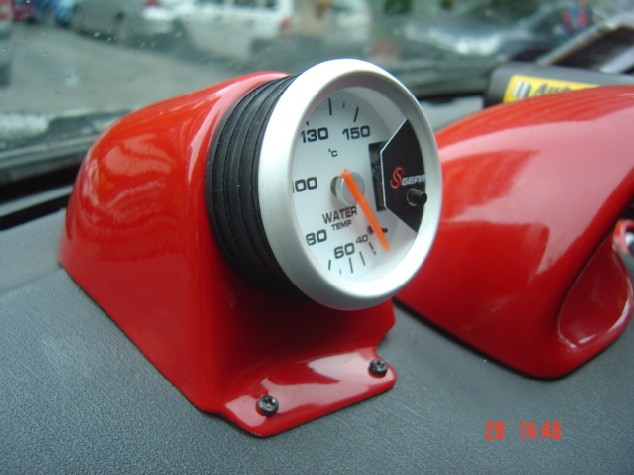In this color photograph taken inside a car, a water temperature gauge is prominently mounted on the dashboard or near the rear window. The gauge features measurements marked at 40, 60, 80, 100, 130, and 150, and is clearly labeled "Water Temp." Next to it rests a curved red metal object. To the right, partially obscured, is a black bottle with a yellow label, its text unreadable.

In the lower right corner of the photograph, the numbers “28” and the time “1446” are digitally displayed. Through the blurry, mist-covered windshield or rear window, several parked vehicles are visible, including a white SUV and a gray van. The overall scene suggests a slightly rainy or misty day.